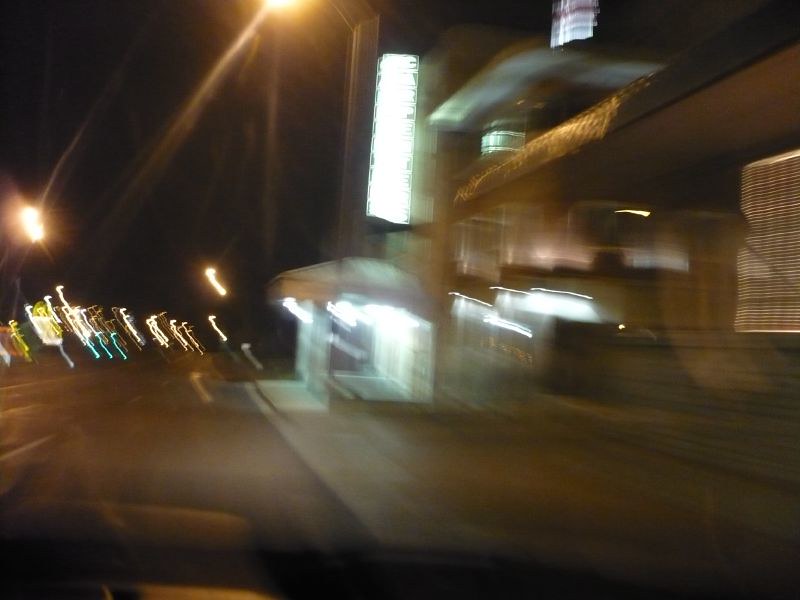The photo, taken at night from a moving car, captures a blurry, horizontally aligned street scene. The image is out of focus, suggesting the viewer is looking through a car window. In the upper left-hand corner, the dark sky is punctuated by yellowish and whitish streetlights mounted on steel poles. Ahead, on the left side of the street, stands a commercial building with an unreadable neon sign above an awning illuminated by lights. The awning area, featuring a small roof that could potentially be a bus stop or entrance, is also blurry with a yellowish hue. The street scene suggests bustling city activity, with additional lights visible further down the road, indicating other parts of the city coming into view.